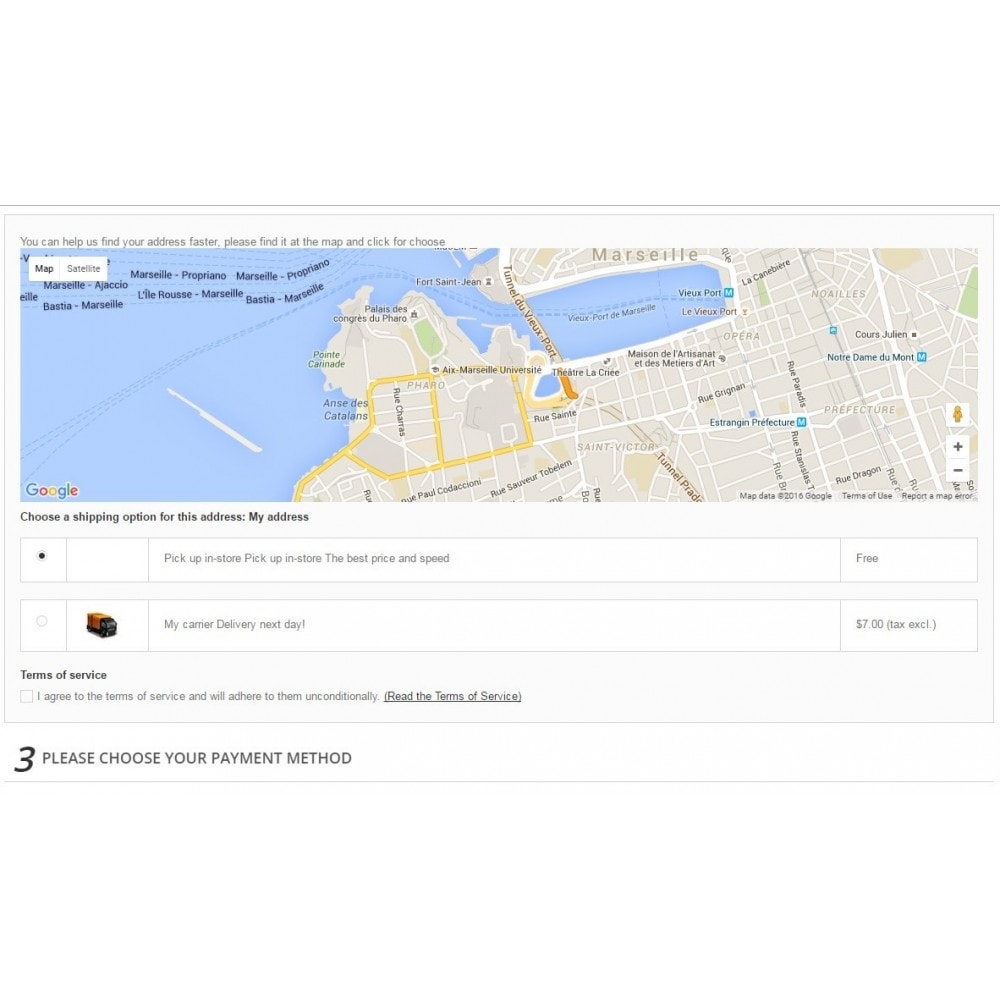Here is the refined and detailed caption:

---

"The web page displays a comprehensive interface with a horizontally-stretched layout. At the top, a gray border contains the message, 'You can help us find your address faster. Please locate it on the map and click to choose.' The interface offers both 'Map' and 'Satellite' views of a location, prominently featuring an image of a map with a large body of water extending into the land. A yellow border outlines a specific section of the map, highlighting various green areas and white side streets. The map is powered by Google, with the Google logo—featuring red, green, blue, and gold colors—visible in the lower right-hand corner.

Beneath the map, instructions prompt users to 'Choose a shipping option for this address.' Several options are presented: 'Pick up in store,' which is noted for offering the best price and speed and is labeled as free, and another option for next-day delivery by a carrier, priced at $7 (tax excluded). There is a mention of the 'Terms of Service,' which users are required to agree to, and they are encouraged to read the terms ('Read the terms of service' is highlighted in bold). Following this, users are instructed to 'Please choose your payment method'—displayed in all caps alongside a numeral three."

---

This caption provides a clear and detailed description of the image, conveying the essence of the web page's layout and functionality.